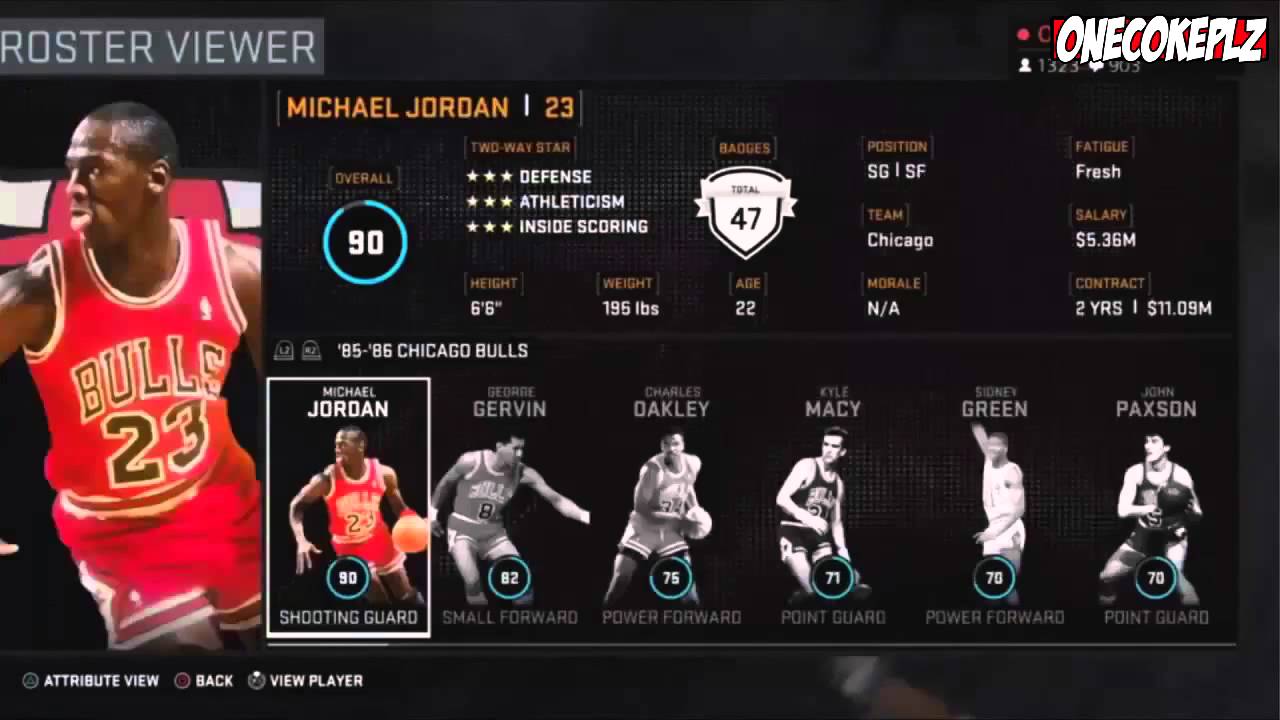Screenshot from Sports Page Depicting Michael Jordan's Player Profile:

The image is a screenshot from an online sports page featuring an extensive profile of NBA legend Michael Jordan. Dominating the left side, a vibrant photograph captures Jordan in action, donning his iconic Chicago Bulls number 23 uniform, with his signature pose—tongue hanging out in concentration. Above this image, the label "Roster Viewer" is prominently displayed, indicating the interactive nature of the page.

To the right of Jordan's image, a detailed breakdown of his statistics and personal information is presented:

- Name: Michael Jordan
- Jersey Number: 23
- Defense: ★★★☆☆
- Athleticism: ★★★☆☆
- Inside Scoring: (stars or additional detail not provided)
- Position: SG/SF (Shooting Guard/Small Forward)
- Team: Chicago Bulls
- Salary: $5.36 million annually
- Contract: 2 years, worth a total of $11.09 million.

At the bottom of this section, there’s a series of smaller player portraits, with Michael Jordan's picture highlighted in full color, indicating it has been selected. The remaining five portraits are in black and white, suggesting unselected profiles. These players are listed as:

1. George Gervin
2. Charles Oakley
3. Kyle Macy
4. Sidney Green
5. John Paxson

This interactive element on the sports page allows users to click on any player’s portrait to reveal their respective information, implying a comprehensive team roster viewer.